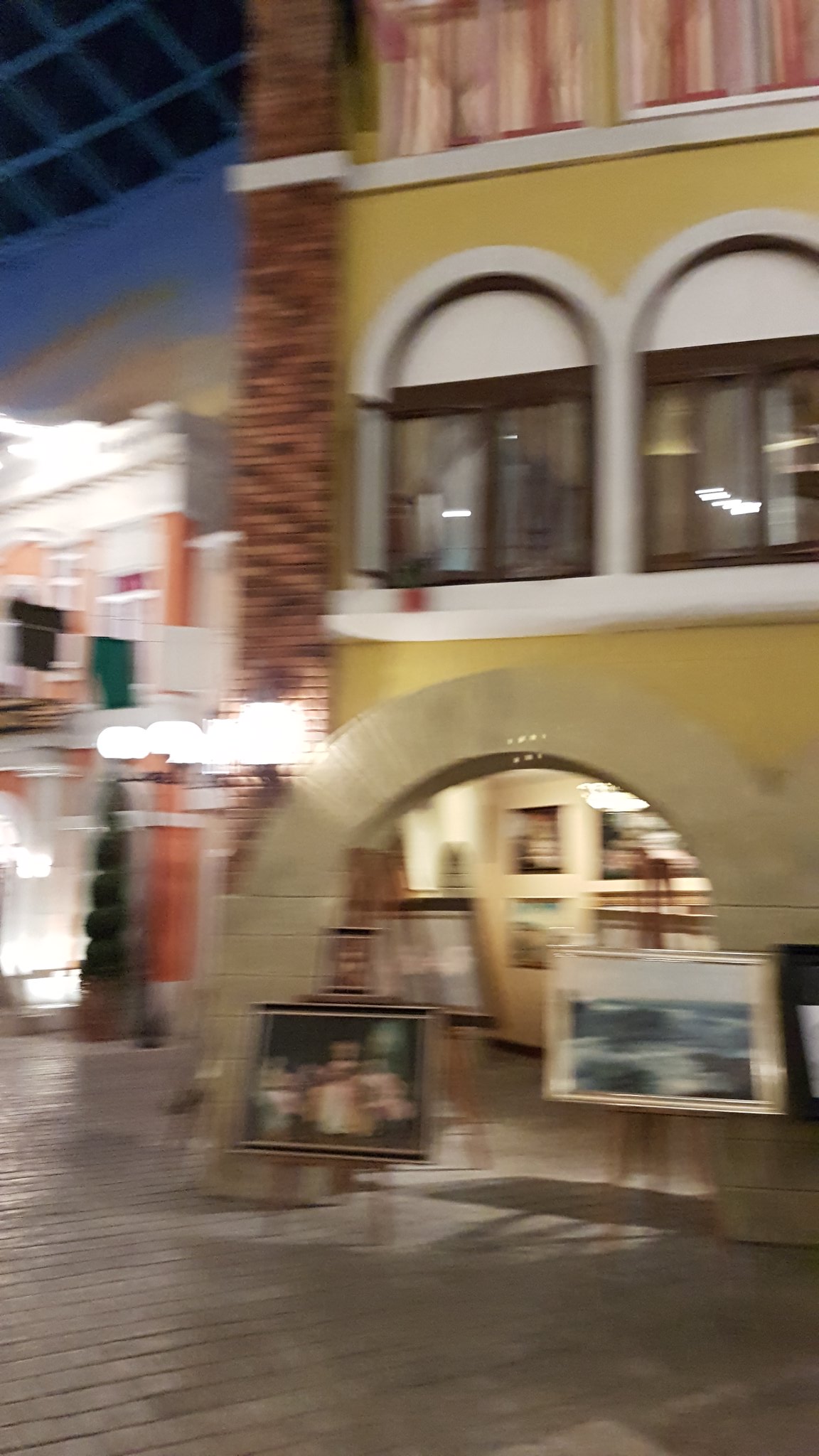The image is a very blurry photograph of a colorful street scene in front of a marigold yellow stucco building. The ground is a gray cobblestone street with some sort of cement divider. Central to the image are several paintings displayed on low easels. One painting depicts a water scene with a white and blue color scheme, while another has a black background with indistinct lighter objects in the foreground. An upside-down U-shaped, or curved, arched entranceway leads into the building, and there are more paintings visible inside. Above the entrance are two square windows framed in white arches with brown trim. The building features defined white concrete floor separators and gray columns. To the left, the photo captures parts of additional buildings, one appearing white and orange, and another with some blue color at the top. Some framed pictures are visible on the building's wall, highlighted by light shining through.